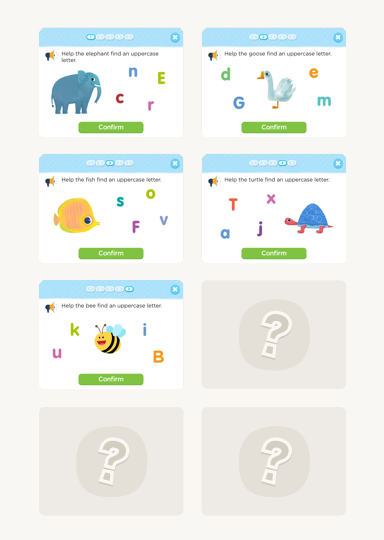Screenshot of a website displaying a puzzle-like interface, featuring an interactive activity designed for children. The main area is a large square grid divided into eight smaller rectangular boxes, arranged in four rows and two columns.

**First Column:**
1. **Top Box:**
   - Blue header bar with an icon and text instructing, "Help the elephant find an uppercase letter."
   - Illustration of a small blue elephant.
   - Letters: "NEC AR"
   - Green "Confirm" button with white lettering.

2. **Second Box:**
   - Similar layout with a yellow fish illustration.
   - Letters: "S O FB"
   - Instructions partially obscured.
   - Green "Confirm" button.

3. **Third Box:**
   - Layout repeated with a happy bee illustration.
   - Letters: "K U I B"
   - Green "Confirm" button.

4. **Bottom Box:**
   - Gray box with a central circle containing a question mark, all in grayscale tones.

**Second Column:**
1. **Top Box:**
   - Blue header bar with an icon, featuring an illustration of a duck.
   - Letters: "D G EM"
   - Green "Confirm" button.

2. **Second Box:**
   - Layout with a blue and red turtle illustration.
   - Letters: "T X AJ"
   - Green "Confirm" button.

3. **Bottom Two Boxes:**
   - Both display gray and white designs with a question mark in the center, indicating inactive or locked sections.

The interface appears to be part of an educational game or activity, with a focus on matching letters or identifying certain letters as prompted by the visual cues and instructions provided in each box.